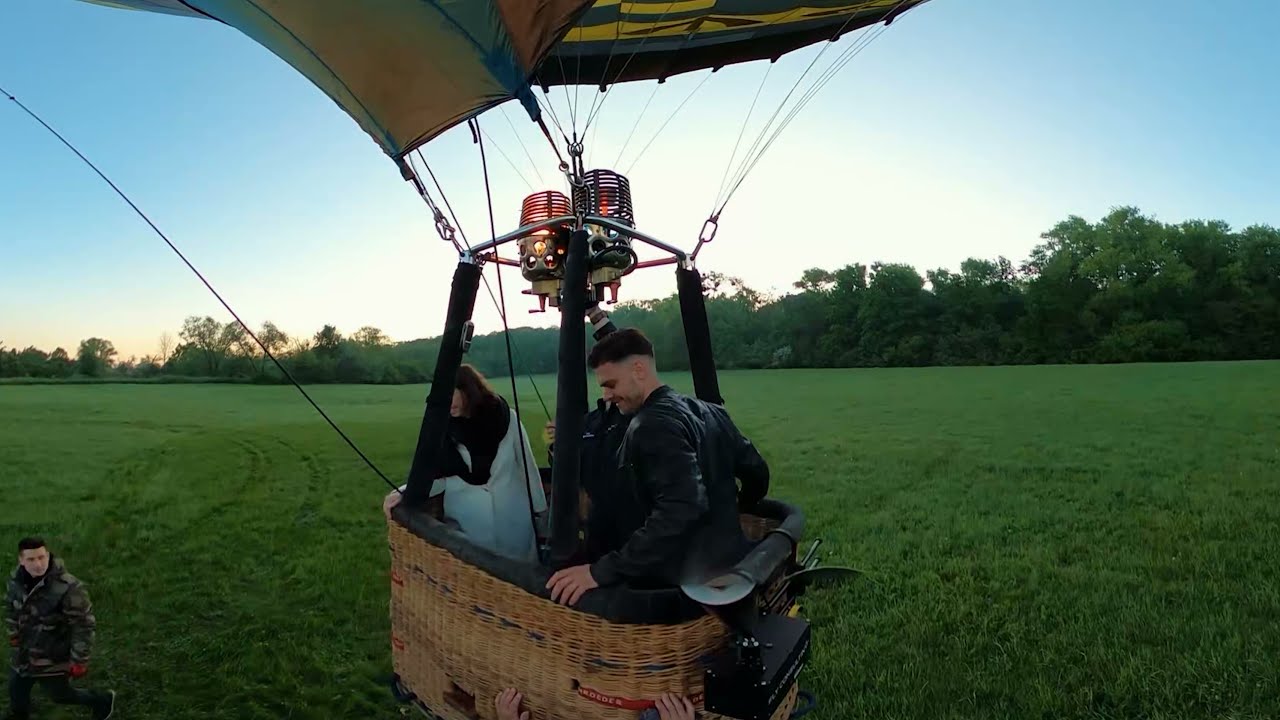The image depicts a hot air balloon in a vast, green grassy field under a mostly clear, blue sky with some white areas, suggesting a sunrise or sunset glow. The balloon itself is shown from the bottom of the basket to just above where the balloon fabric starts, revealing its multicolored design. Inside the basket, there are three people: a man wearing a black leather jacket with short black hair shaved on the sides, a woman with brown hair in a long white jacket with black trim and possibly a black scarf, and another man mostly hidden behind the first man, presumed to be operating the controls. A fourth person, clad in a camouflage jacket, is seen in the bottom left corner, close to the ground and inspecting the balloon. The background features a line of green leafy trees several hundred feet away, contributing to the serene atmosphere of the outdoor setting. The heating mechanism under the balloon is visible, indicating the balloon may be just about to take off or hovering slightly above the ground.